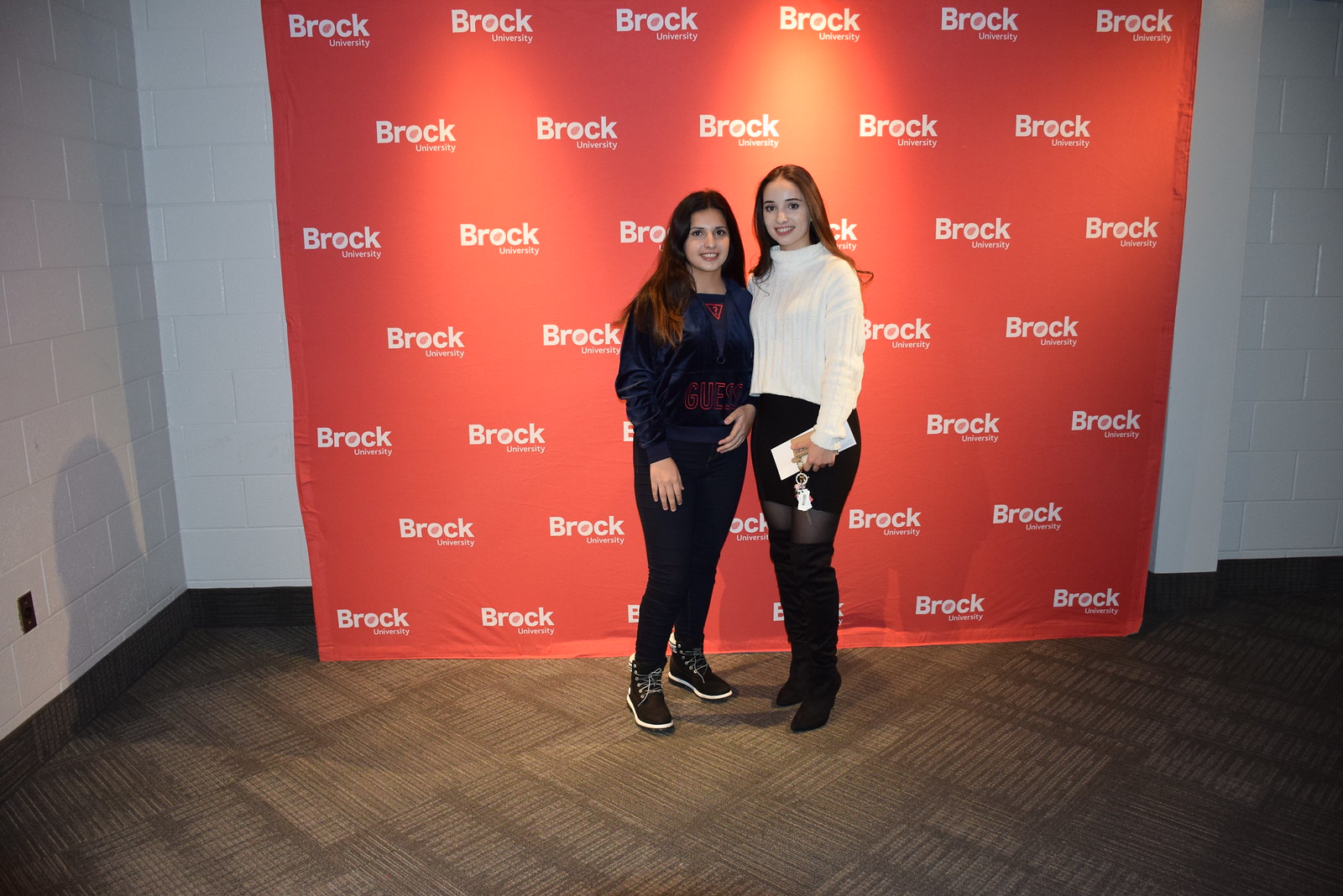This image showcases two young women standing side by side in an indoor setting, posing in front of a red promotional backdrop featuring the words "Brock University" repeatedly in white. Both appear to be around 15 or 16 years old, likely of Caucasian descent. The girl on the left has long, dark brown hair with lighter highlights and wears a dark navy blue top with red text that says "Guess", paired with black jeans and black-and-white boots. Her posture is slightly angled towards her friend, with her face turned towards the camera and her left arm seemingly bent at the elbow. The girl on her right has light brown hair and is dressed in a white turtleneck sweater, a black skirt over black nylons, and knee-high black boots. She holds what looks like a book and a set of keys in her left hand, with her right arm relaxed at her side. The red display wall they stand before appears to be over a brown carpet, with the surrounding walls painted white.